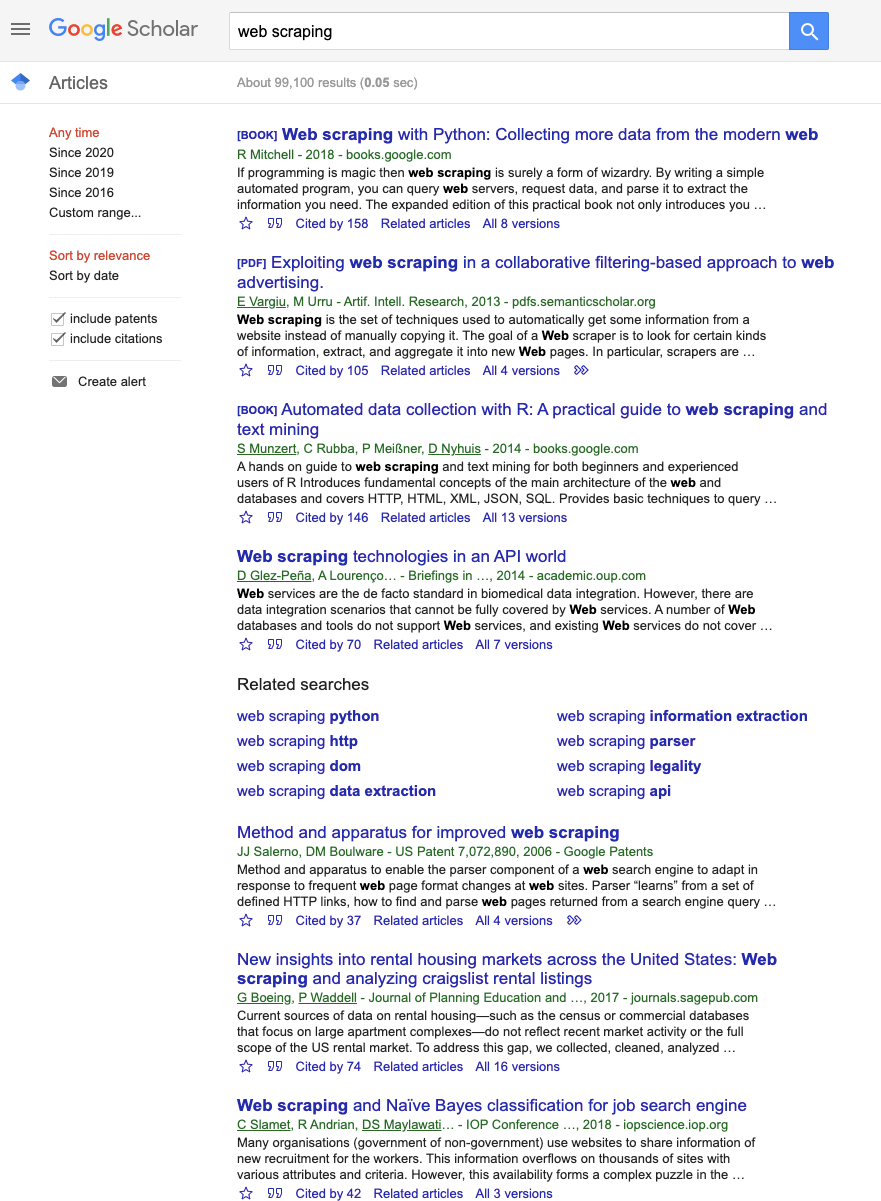The image displays a Google Scholar search results page. In the top left corner, the logo clearly reads "Google Scholar." A search query, "web scraping," is typed into the search box located at the top of the page. Below the search query, a series of results are prominently listed.

1. The first result is a book titled "Web Scraping with Python: Collecting More Data from the Modern Web," complete with the author's name and detailed book information.
2. The second result is a PDF titled "Exploiting Web Scraping in a Collaborative Filtering-Based Approach to Web Advertising," which includes the author's name, the publication year, and additional details about the document.
3. The third result is another book titled "Automated Data Collection with R: A Practical Guide to Web Scraping and Text Mining." This entry lists multiple authors and provides further details about the book.
4. The fourth result is an article titled "Web Scraping Technologies in an API World," accompanied by the author's name and specific publication details.
5. Following these initial entries, there is a section of related searches.
6. Below this section, another article appears, titled "Method and Apparatus for Improved Web Scraping," along with the names of the authors and publication details.
7. Further down, another result is visible: "New Insights into Rental Housing Markets Across the United States: Web Scraping and Analyzing Craigslist Rental Listings."
8. The final search result listed is "Web Scraping and Naive Bayes Classification for Job Search Engine."

Each entry lists the title, author(s), and additional publication details, providing a comprehensive overview of scholarly works related to web scraping.